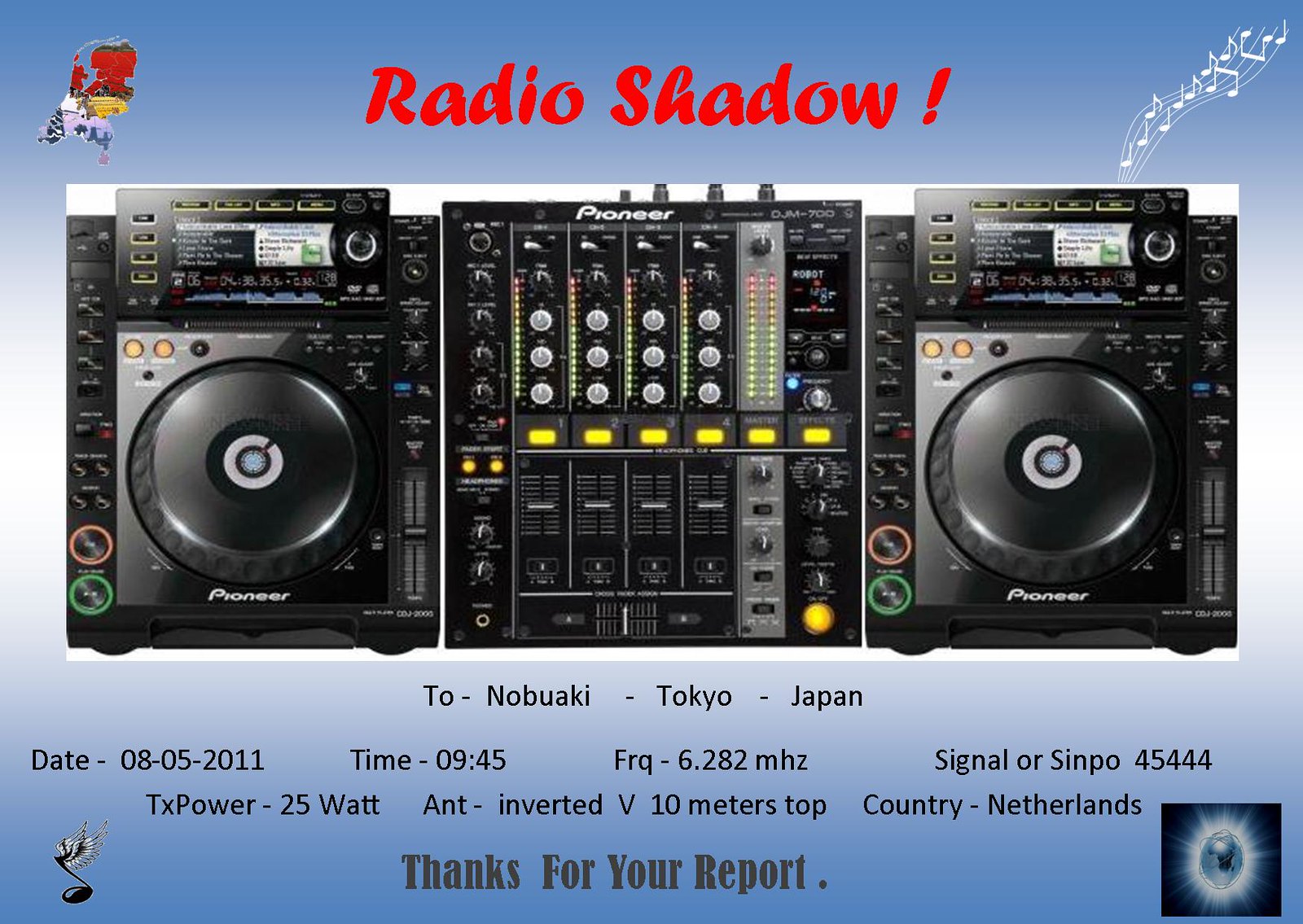The advertisement titled "Radio Shadow!" features a vast and detailed stereo system made by Pioneer, prominently displayed against a blue background. The stereo system appears to be a three-piece setup with an equalizer flanked by two large speakers. The equipment is festooned with multiple buttons and dials in various colors—white, red, yellow, and green—with a noticeable stream of lights cascading from the top right toward the middle. Cartoon music notes emanate from the top right speaker, enhancing the dynamic and lively feel of the ad. 

Below the image of the stereo system, black text reads: "TOE-NOBUAKI-TOKYO-JAPAN." This is followed by detailed information including the date "08.05.2011," time "09.45," frequency "6.282 MHz," signal "SINPOE: 45444," transmission power "25 watts," antenna type "Inverted V, 10 meters top," and the country "Netherlands." The bottom of the flyer expresses gratitude with "Thanks for your report." Additional graphic elements include a musical note in the lower left corner and a starburst in the right corner, both set against a dark blue background.